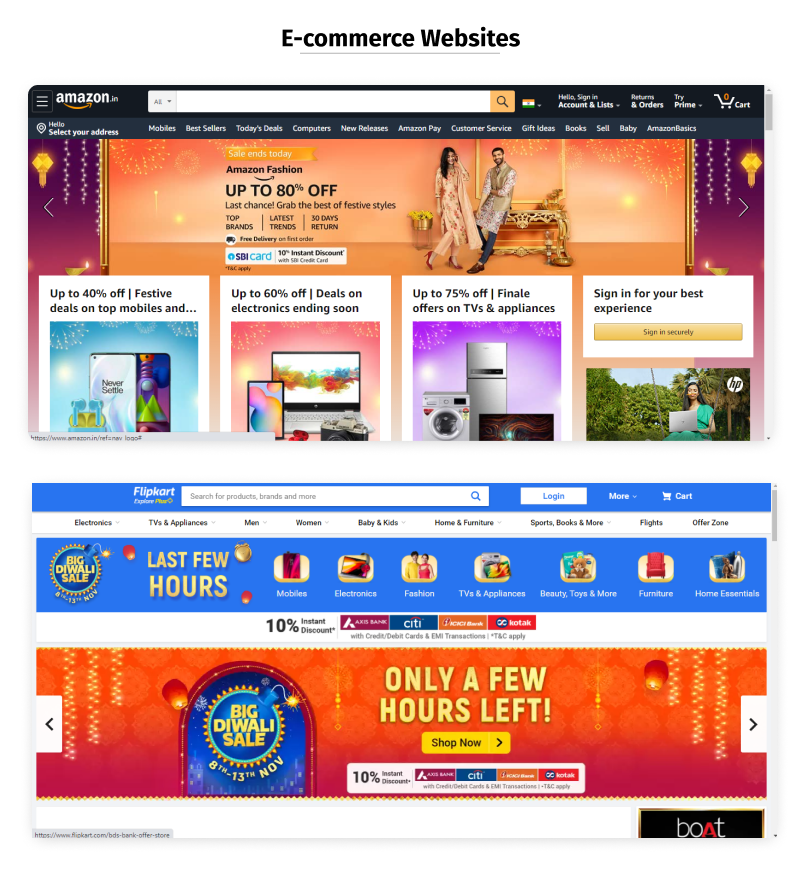**Description of the Advertisement:**

The advertisement is from Amazon, showcasing various e-commerce features and ongoing sales. At the top of the image is a black bar with the Amazon logo situated in the right corner, alongside a swirling arrow pointing from 'A' to 'Z'. This bar includes options like "Sign-in Account," "Delivery and Orders," and indicates there is one item in the cart.

Below this, there's another toolbar displaying several categories: "Hello, Select Your Address," "Mobile," "Bestsellers," "Today's Deals," "Computers," "New Releases," "Amazon Pay," "Customer Service," "Gift Ideas," "Books," "Sell," and "Babies and Accessories."

An orange banner features prominently, depicting two people standing against some furniture. This banner advertises Amazon Fashion with up to 80% off under a "Last Chance Grab the Best of Festive Styles" promotion. It highlights top brands and latest trends with a 30-day return policy, mentioning free delivery on the first order and a 10% instant discount for SBI card users.

Below this banner, four square sections showcase various deals:
1. **Mobile Deals:** Featuring an iPhone with up to 40% off on festive deals on top mobiles.
2. **Electronics Deals:** Displaying a laptop, camera, and phone, offering up to 60% off on electronics with deals ending soon.
3. **Appliances Deals:** Highlighting a washer, refrigerator, and TV, promoting up to 75% off on final offers for TVs and appliances, with a prompt to sign in for the best experience.

Further below, a blue toolbar from Flipkart presents different sections such as "Login," "More," "Cart," "Electronics," "TVs and Appliances," "Men," "Women," "Baby and Kids," "Home and Furniture," "Sports," "Books and More," "Flights," and "Offers." Each of these sections has a corresponding icon.

At the bottom, another orange banner announces the "Big Diwali Sale" from November 8th to 13th, emphasizing that only a few hours are left to shop. This includes a 10% discount, urging customers to take advantage of the sale immediately.